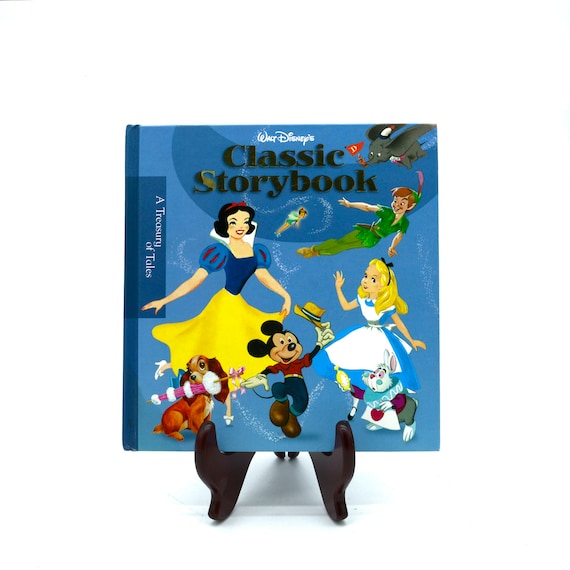This image features a vintage Walt Disney classic storybook, likely from the late 1960s to early 1970s, displayed on a brown stand. The book's predominantly blue cover prominently features "Walt Disney" in Disney's iconic font at the top, with "classic storybook" written in large black letters underneath, split onto two lines. On the right, a dark blue rectangle with white lettering proclaims "A treasury of tales," oriented perpendicularly to the title.

The cover is adorned with beloved Disney characters in a delightful arrangement. At the top left, Dumbo the flying elephant swoops downwards with a small mouse on his trunk, holding a red flag bearing a yellow 'D.' Below Dumbo is Peter Pan in his green outfit, complete with a hat and feather, and to his right, Tinkerbell hovers, spreading pixie dust over the scene. Snow White stands near the center-right, looking radiant with her red bow, black hair, fair skin, classic blue and yellow attire, and a friendly smile. In the bottom right corner, Lady, the Cocker Spaniel from "Lady and the Tramp," is depicted charmingly with a pink and white frilly umbrella in her mouth. Central to the composition is Mickey Mouse, donning his iconic red shirt, blue pants, and brown shoes, holding his cap with a cheerful expression. To Mickey's left stands Alice from "Alice in Wonderland," with her blonde hair and traditional blue dress. In the far left corner, the White Rabbit from the same story can be seen, holding his timepiece and gazing towards Mickey. The entire cover is brought to life with Tinkerbell's magic dust, adding an enchanting sparkle to this nostalgic and colorful assemblage of Disney characters.